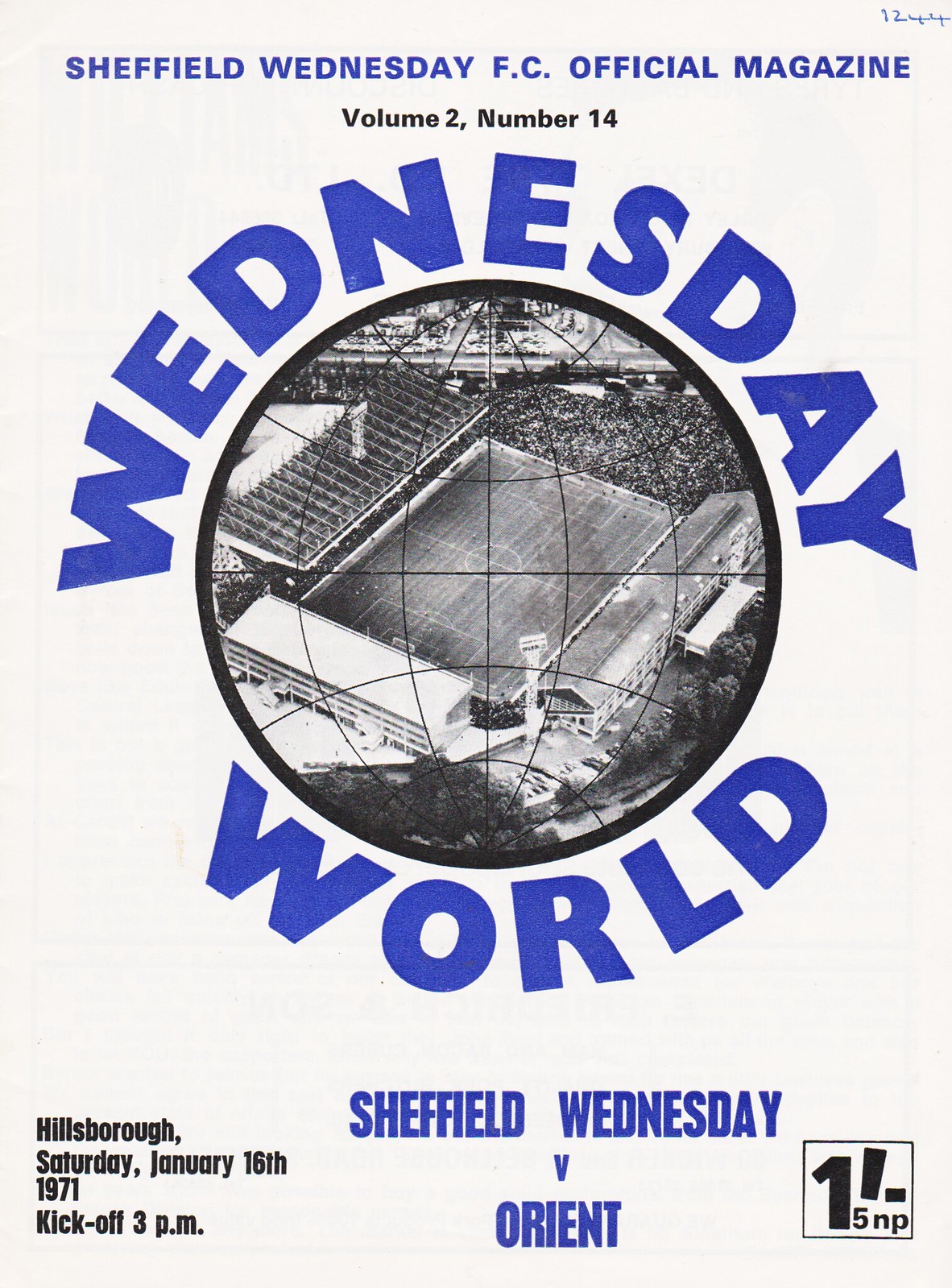The image is a magazine cover predominantly featuring a solid white background with text from the next page faintly visible through it. At the very top, handwritten in blue ink are the numbers "1244," followed by the title in blue text: "Sheffield Wednesday FC Official Magazine." Beneath this, in smaller black text, it reads "Volume 2, Number 14." Centrally positioned on the cover is a globe, superimposed over an aerial view of a black and white photograph of a soccer field. Encircling this globe in large blue font are the words "Wednesday World." At the bottom of the cover, three lines of text in blue font read "Sheffield Wednesday V Orient." Additionally, the bottom left corner specifies "Hillsborough Saturday January 16, 1971, Kickoff 3 p.m." A square symbol in the bottom right corner displays "1 / 5 P."